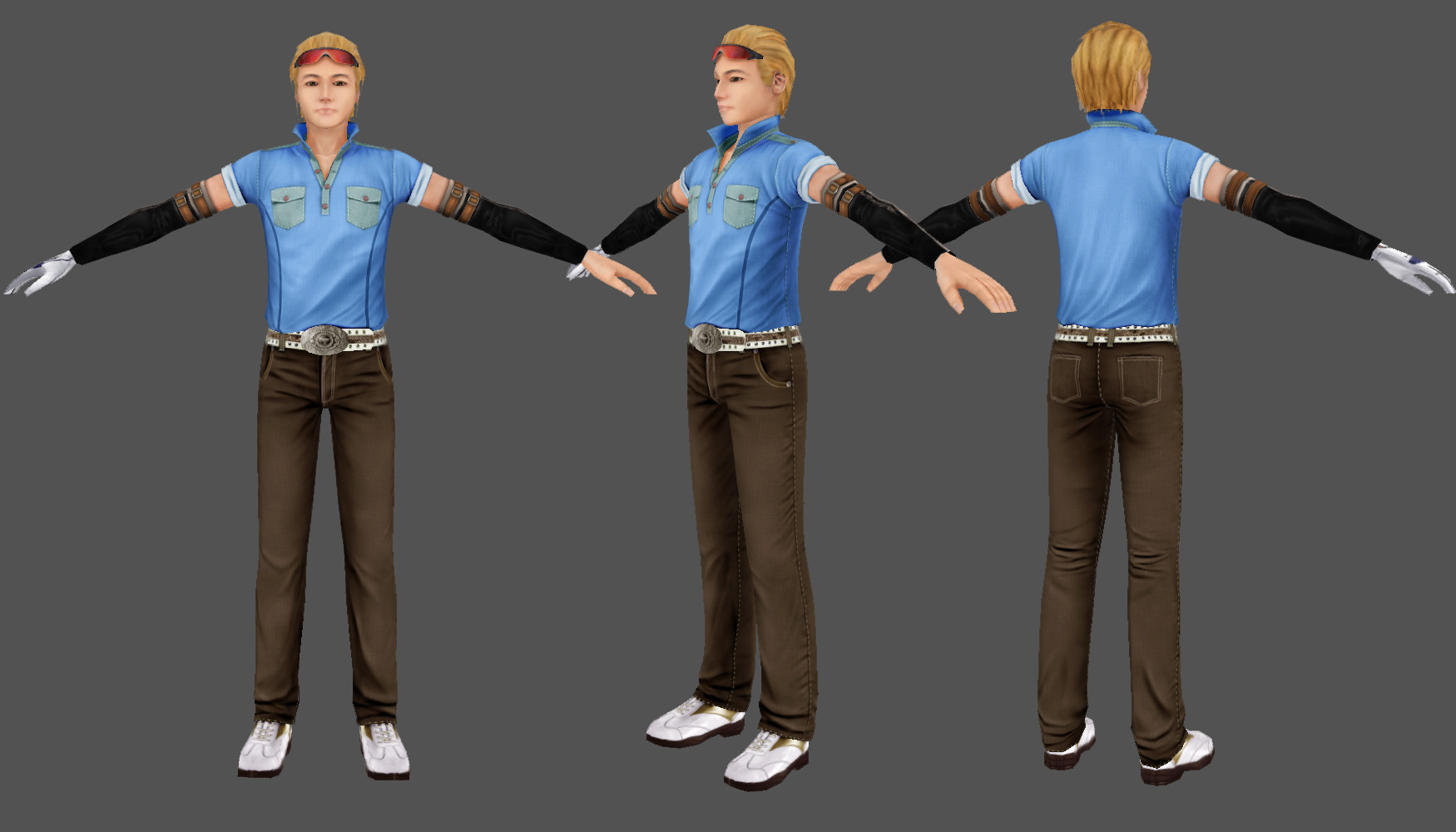The image showcases a 3D-rendered androgynous cartoon character depicted three times in identical poses but from different angles—front, left side, and back view—appearing to be mid-turn. The figure has short blonde hair and wears red sunglasses perched on the forehead, emphasizing a casual yet distinctive style. They are dressed in a blue polo shirt with two chest pockets, black detached sleeve cuffs, and black jeans, secured with a white and brown belt that features a silver buckle. The character's right hand is adorned with a white glove, and they sport white sneakers with black heels. Each rendition of the character overlaps at the arms, which are spread out to the sides. The background is predominantly gray with a darker gradient around the edges, emphasizing the three-dimensionality of the render.